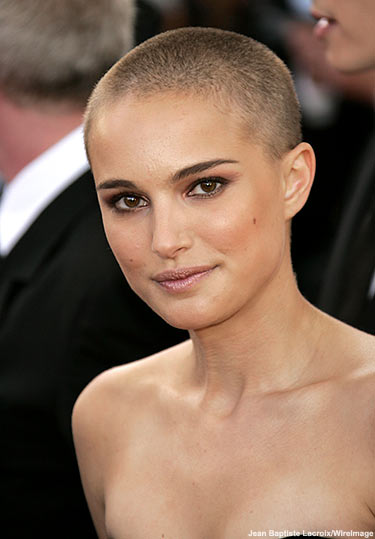This is a detailed close-up photograph of a young Natalie Portman, taken from the chest up. She is almost bald with her hair shaved extremely short, reminiscent of her appearance during the filming of "V for Vendetta." Natalie is wearing a strapless or sleeveless dress, although only a small portion of it is visible. Her makeup includes a touch of eyeshadow, mascara, and a light pink or beige-toned lipstick. She has dark brown hair and brown eyes, with well-groomed eyebrows. Natalie is looking directly at the camera, and her face has a slight sheen indicative of makeup. In the blurry background, there are at least two other individuals: a man in a suit with a white collared shirt and grayish hair, and another person possibly in a black outfit. The setting suggests that this could be a red carpet event or movie premiere. In the bottom right corner of the image, there is small, hard-to-read white text that credits "Jean-Baptiste Lecroix / WireImage."